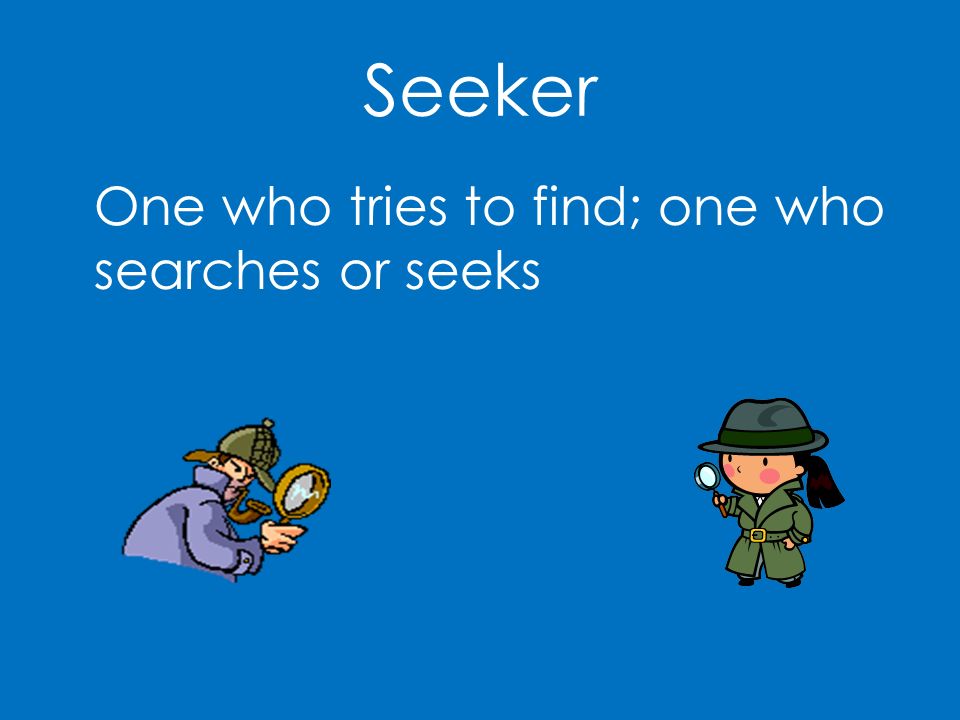The image, set against a darker blue background, features prominently centered white text that reads "SEEKER" with a capital "S" at the top. Directly below this headline, also in white text but slightly smaller, is the definition: "one who tries to find; one who searches or seeks." Beneath the text, the image is divided into two sections. On the left side, there's a retro, computer graphic-style depiction of a male detective reminiscent of Sherlock Holmes. He dons a deerstalker cap and a purple trench coat, has a pipe in his mouth, and holds a large magnifying glass in his right hand, looking through it intently. On the right side is an animated female detective. She has black hair with a ponytail, wears a green trench coat with a gold belt buckle, a matching hat, and black boots. Her cheeks are faintly blushed, and she also holds a magnifying glass in her right hand, peering through it. The overall design of the poster or slide emphasizes the concept of a "seeker" as someone engaged in the act of searching and discovering.